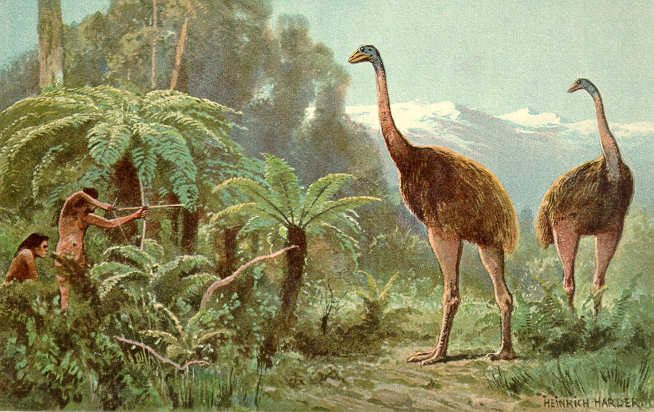The illustration appears to be a detailed artist's rendering set in prehistoric times, possibly intended for a book. It depicts a lush, tropical forest filled with various types of greenery, including ferns, grasses, and short palm-like trees. In the foreground, two human-like creatures are engaged in a hunt. The primary hunter, standing upright and naked, is poised with a bow and arrow aimed at two massive, ostrich-like birds. These birds are about twice the height of the humans, with long necks, bare legs, and furry feathers but no wings for flying, resembling modern-day emus but significantly larger. Crouched behind the primary hunter and partly hidden in the dense foliage is a second hunter with long hair, also nude. In the distant background, snow-capped mountains rise above the horizon, enhancing the scene's prehistoric and wild atmosphere.